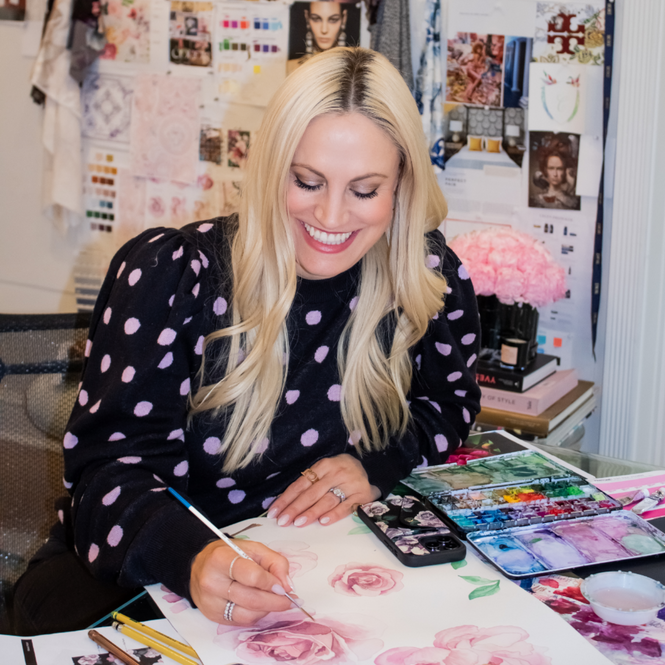In this detailed photograph, a young woman with long platinum blonde hair, with her roots showing, is captured in a moment of creative joy as she paints watercolor flowers. Dressed in a black outfit adorned with pink polka dots, she smiles warmly, revealing her teeth, while focusing intently on the artwork before her. Her right hand delicately holds a paintbrush above a piece of paper where she is painting pink roses or carnations. In her left hand, she steadies the paper. Scattered around her workspace are several art supplies: a palette of watercolors and three pencils (two yellow and one brown) to her right, and in front of her, a small bowl of water. A phone lies face down next to her, its case decorated with pink flowers. Behind her, an inspiring bulletin board displays photographs of people, fashion, and various color palettes, echoing her artistic endeavors. Adding a touch of life to the scene, a vase of pink flowers, similar to those she is painting, stands triumphantly in the background, blending the real with the depicted. Her room, a cozy sanctuary filled with artistic inspiration, sets the perfect backdrop for this intimate and lively portrait of a dedicated artist.